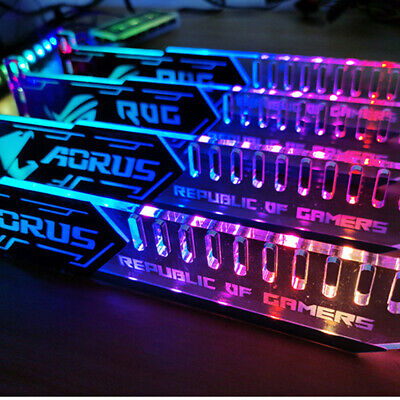The photograph showcases four pieces of acrylic computer equipment lined up in a row, set on a black surface. Each piece features a black handle with stylized lettering; two of them read "Aorus", while the others display "RUG". Below the handles, an inscription of "Republic of Gamers" is clearly visible. The top edges of these objects transition from turquoise to a spectrum of vibrant LED colors—blue, pink, red, and yellow—that seemingly glow without a visible light source, creating a captivating neon effect. The oblong shapes and big, comb-like enclosed teeth suggest they might organize or hold computer wires. The backdrop enhances the scene with a subtle purple illumination, hinting at a sophisticated setup, possibly a gaming or tech-oriented workspace.